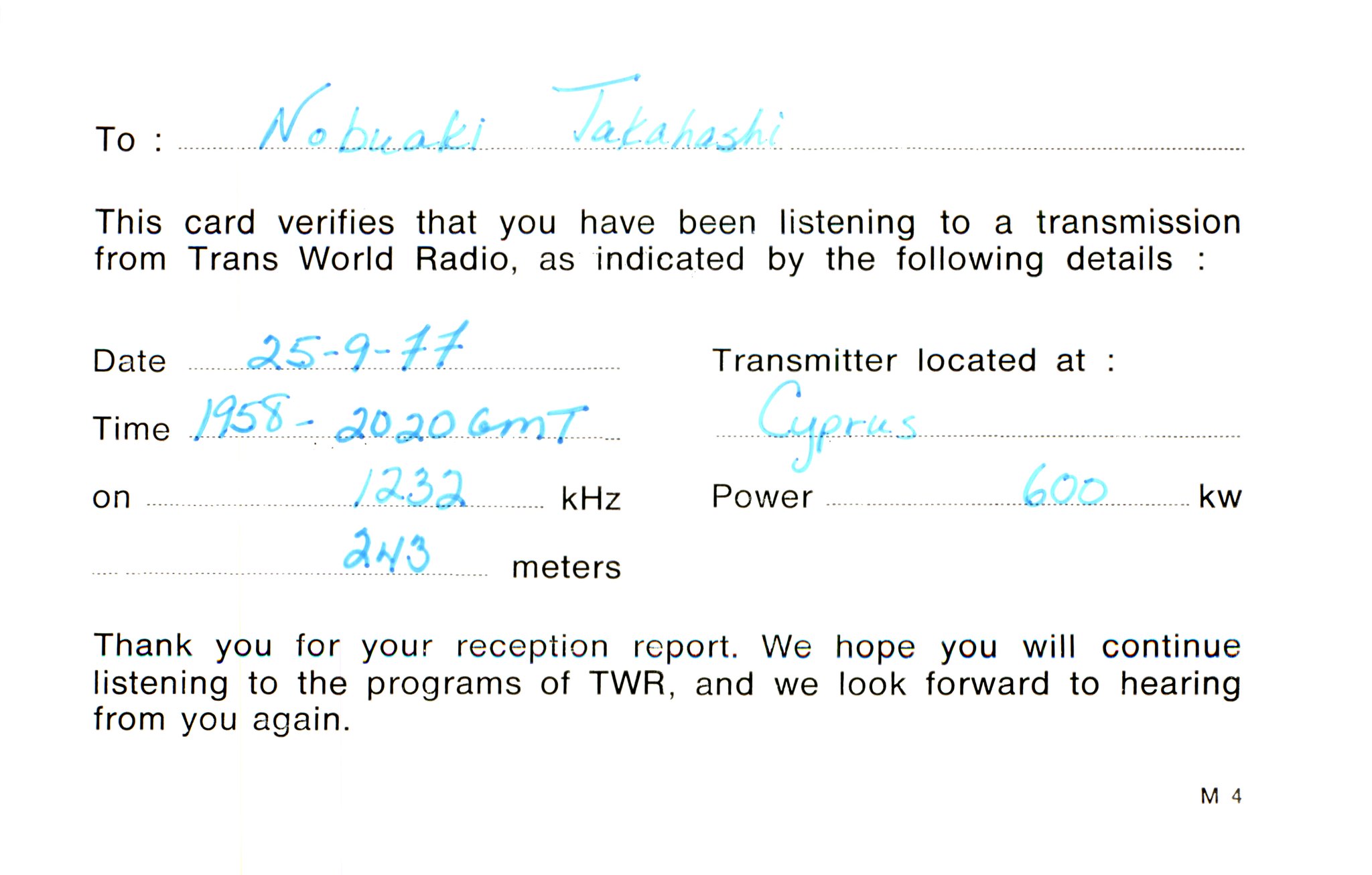The image is a black-and-white card with both typed and handwritten text. A key part of the card includes handwritten entries in blue ink. The typed text starts with "To:" followed by the blue handwriting "Nobuaki Takahashi." Below that, the card states, "This card verifies that you have been listening to a transmission from Trans World Radio as indicated by the following details." In blue ink, the date "25-9-77" is written, followed by the time "1958-2020 GMT," the frequency "1232 kilohertz," and the wavelength "243 meters." The card specifies the transmitter's location at "Cyprus" and states its power as "600 kilowatts." Concluding the card, the typed text reads, "Thank you for your reception report. We hope you will continue listening to the programs of TWR and we look forward to hearing from you again."